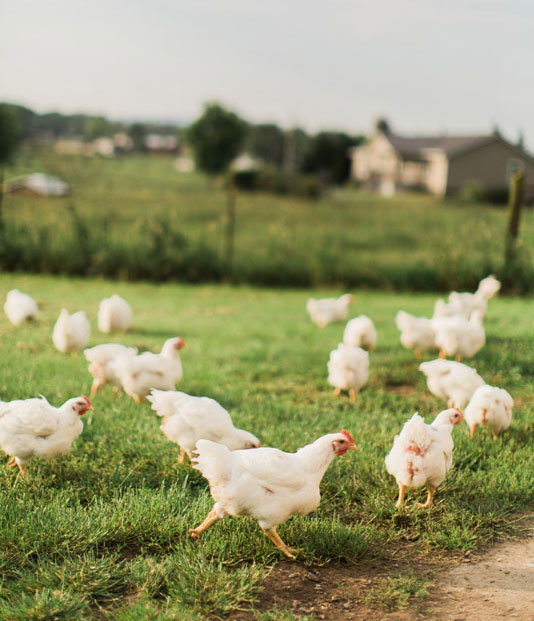The image depicts a lively farm scene centered around a flock of medium-sized, white chickens with distinctive red crests and yellow beaks, walking and grazing on a lush green grassy area. The chickens, over a dozen in number, are all of the same breed with orange legs and curved orange beaks. One prominent chicken stands out in the center of the image, capturing the viewer's primary attention. In the bottom right corner of the foreground, a patch of compact dirt is visible. In the background, there's a blurry but discernible rustic setting that includes a wooden fence made of branch or log posts, possibly with barbed wire, separating the grazing area from taller grass fields beyond. Behind the fence, there are multiple buildings. On the right side, a multi-storied stone house with a grey triangular roof and light brown walls can be seen, while additional structures are located towards the left. The predominant colors in the image include the vivid green of the grass, the white feathers of the chickens, the red of their crests, and the earth tones of the houses and background elements.